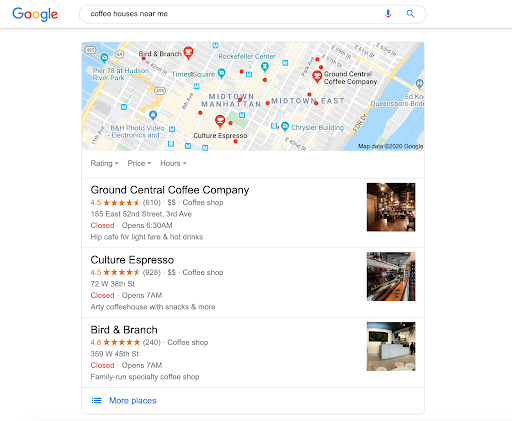The image captures the Google search results for "coffee houses near me," conducted in New York City. At the top of the page, the search bar, prominently displayed in the upper center, clearly indicates the query. Below the search bar, a light gray separator bar delineates the transition to the main content. 

A detailed map takes center stage, highlighting various locations within Midtown Manhattan. Key landmarks such as Midtown East, Rockefeller Center, and Hudson River Park are visible. The map is well-centered, offering a clear overview of the vicinity.

Below the map, the first search result lists Grand Central Coffee Company, boasting a rating of 4.5 stars and an opening time of 8:30 AM. Following that is Cultural Espresso, and the last listing is Burden Branch. The image effectively conveys a comprehensive and detailed presentation of the search results for coffee houses in Midtown Manhattan.